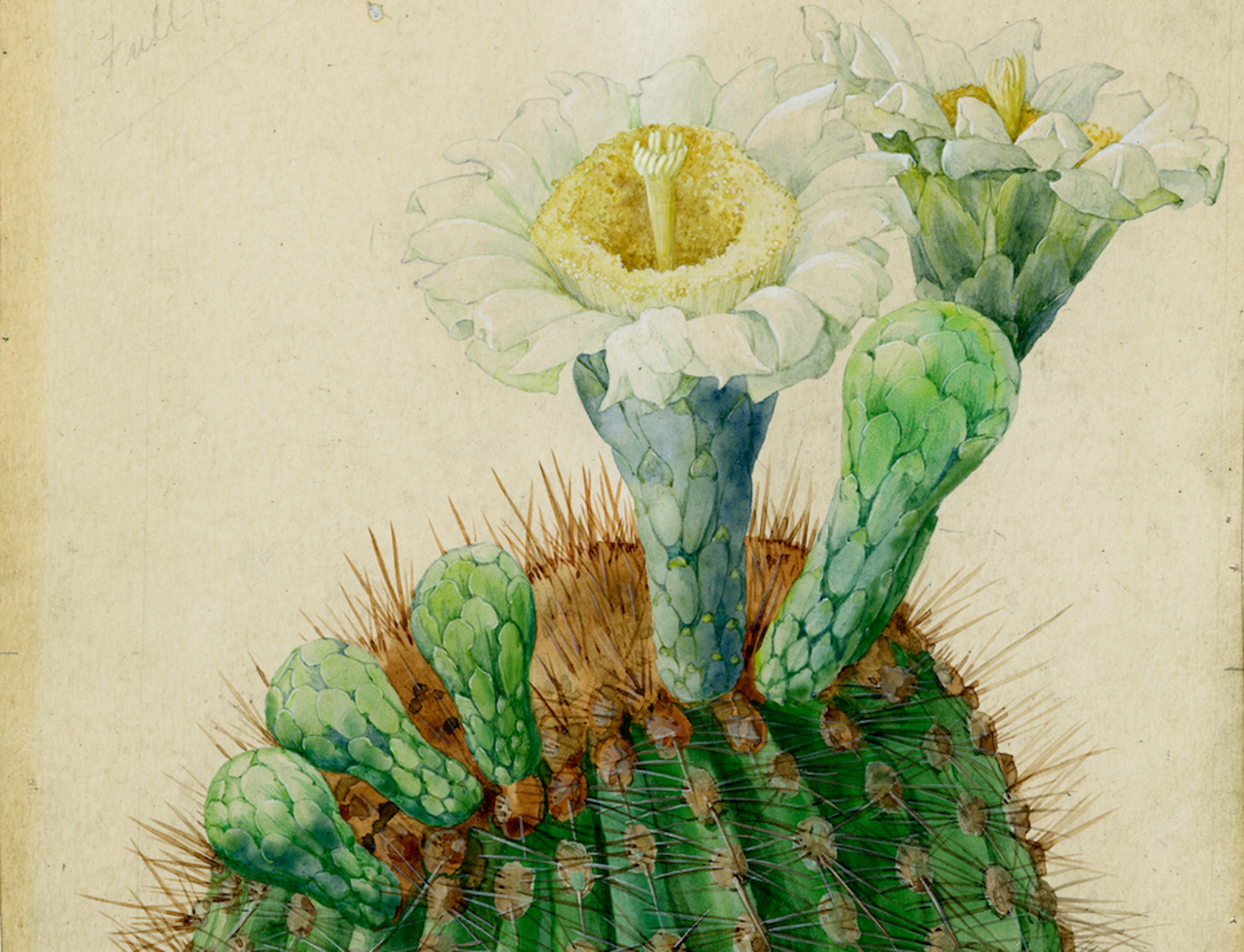This detailed watercolor artwork portrays a blooming cactus set against a textured, yellowish-orange paper, which simulates old, noise-speckled parchment with brownish spots. The cactus itself is robust and green, accentuated with brown spines, and presents a mass of rounded, ribbed domes at the base. The ribs of the cactus, described with a corduroy-like appearance, are lighter at the points where the sharp quills emanate.

From the main body of the cactus, three smaller green protrusions rise on the left, each with a scaly pattern reminiscent of snake skin. At the center of the cactus, a prominent, segmented blue-green protrusion ascends, leading up to a strikingly detailed flower. This flower has white petals encircling a yellow center, and features delicate white stamens.

To the right, another large, bulbous green protrusion reaches upward, comparable in height to the central flower. This section also hosts another blooming flower similar to the central one, with white petals and a yellow center, nested within a fuzzy, brownish cup.

Overall, the artwork captures the intricate details of the cactus in bloom, highlighting the contrast between the textured backdrop and the meticulously detailed cactus and its flowers.